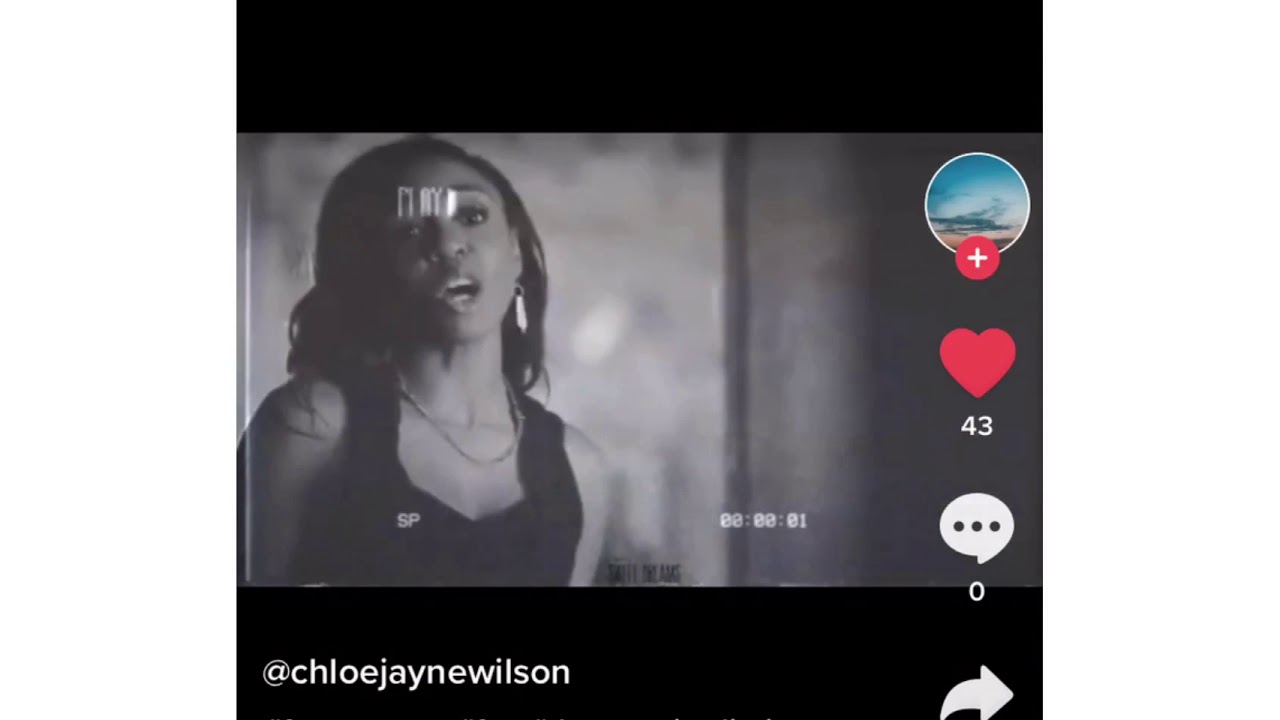This image portrays a young girl who appears to be singing passionately. She is dressed in a stylish square-neck top and has long, black hair. Completing her look, she is adorned with feather-like earrings. The background of the image is a soft, blurry gray, adding a muted yet fitting contrast to her lively expression.

Overlaying the image are several graphic elements. On one side, there is a red "plus" symbol paired with a smaller image of a sunset. Below this, there is a red heart symbol followed by the number 43, indicating likes or favorites. Further down, a message icon with a count of zero is visible alongside a curved arrow symbol, suggesting options for sharing or resharing the image.

These icons and text are enclosed within a black box that contrasts with the blurred gray background. Additionally, the text "@ChloeJJaneWilson" is prominently displayed, likely indicating the girl's social media handle.

On her face, there appears to be a doodle resembling a peculiar "M" and "A" forming the word "May," subtly drawn and adding an unexpected artistic element to the image.